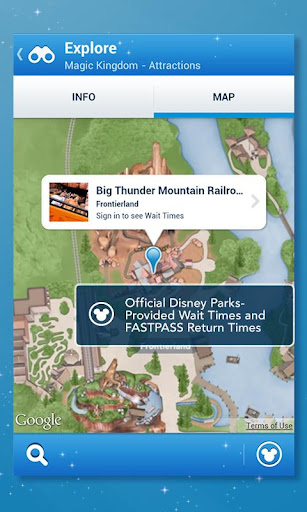Here's a meticulously detailed caption for the image described:

---

**Screenshot of a Theme Park App Interface**

The image is of a theme park application mock-up, resembling what one might see in the Google Play Store or Apple App Store. The background is a rich, dark blue adorned with small, white star-like speckles. These stars extend to the dark blue bezel located at the top and bottom of the application's screenshot, blending seamlessly.

**Top Section: Navigation and Title**
At the top left corner, inside the dark cyan-blue bezel, there's a faded white leftward arrow. Adjacent to it is a pair of white binoculars, featuring dark blue front lenses. To the right, in bold white text, the word "Explore" is prominently displayed. Subtly below, in regular white text, it reads "Magic Kingdom-Attractions."

**Tab Navigation**
The interface has two navigation tabs. The tab on the right, labeled "Map," is highlighted, indicating its selection with a blue band underneath it. The unselected tab, labeled "Info," is in bold black, all capitalized, and appears slightly raised against a light gray background.

**Interactive Map Display**
The main section showcases a detailed map. The map depicts lush green grass and multiple kingdoms and buildings in shades of tan and brown. Light tan, almost cream-colored roads traverse the map, with a notable island on the right connected by a broad bridge to another island. The water bodies are light blue with darker blue edges for contrast.

**Pop-up Information Box**
A white pop-up box with orange bands highlights a specific location. Inside, black text reads "Big Thunder Mountain Railroad," followed by a cut-off section and "Frontierland" beneath it. The pop-up prompts users in gray text to "Sign in to see wait times," accompanied by a dark blue pin.

**Footer Information and Design**
At the bottom, a dark blue rectangle with a white border features the Disney logo—three circles forming the iconic Mickey Mouse shape. The accompanying white text reads: "Official Disney Parks – provided wait times and FASTPASS return times." 

On the lower bezel, the left corner displays "Google" in white text. The right corner houses an opaque white rectangle with bold black, underlined text that says "Terms of Use." Additionally, the lower left side has a bold white magnifying glass icon, while the right side features the Mickey Mouse logo.

---

This detailed caption encapsulates every visual element and intricate detail described in the voice note.